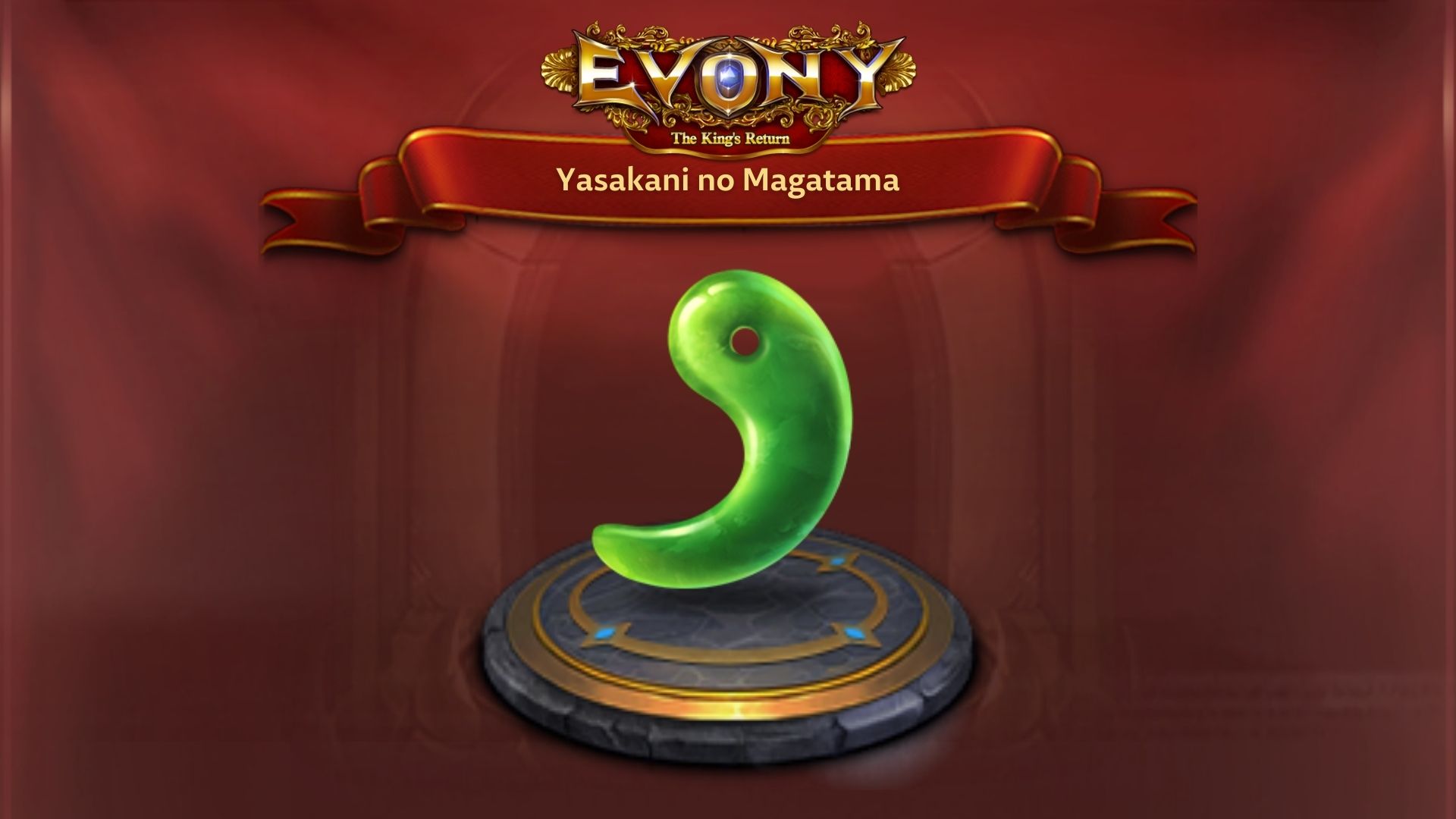This image shows a game loading screen labeled "Evony: The King's Return." At the top, "Evony" is written in gilded gold letters, with intricate symbols surrounding it, and the 'O' illuminated with a bluish light. Beneath it, "The King's Return" is displayed. Below this, a crimson ribbon with a gold outline bears the inscription "Yasakani no Magatama" in gold lettering. Central to the image is a prominent green, semi-circular yin-yang symbol, positioned above a charcoal stone platform with two concentric gold borders. Within the inner gold border, three visible diamonds are embedded. The background is a transparent red, revealing the entrance to an ancient tomb or hallway, enhancing the exotic and historical ambiance of the scene.